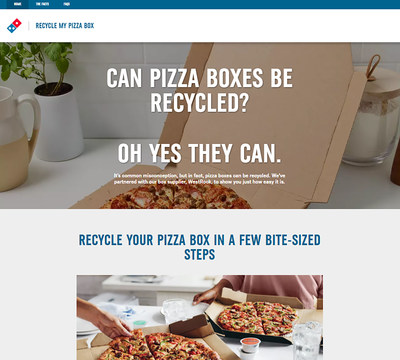This is a screenshot taken on a desktop or laptop computer featuring the Domino's Pizza website. The website's navigation bar includes several buttons, with legible ones being "Home" and "Menu," though the resolution is low and some text appears blurry. Beneath the navigation bar, there is a prominent white banner with blue text that reads, "Recycle My Pizza Box." The Domino's logo is displayed to the left of this banner; the logo is designed as a red and blue domino featuring three dots.

Directly below, another banner prompts the question "Can Pizza Boxes Be Recycled?" followed by the affirmation, "Oh yes they can." This is accompanied by an image showcasing a Domino's pizza in an open cardboard box resting on a white table. The text beneath this image states, "Recycle Your Pizza Box in a few bite-sized steps."

Further down the page, there is a photo of two individuals enjoying their Domino's pizza from the boxes. The webpage serves as an informational guide encouraging users to recycle their Domino's pizza boxes instead of discarding them in the trash.